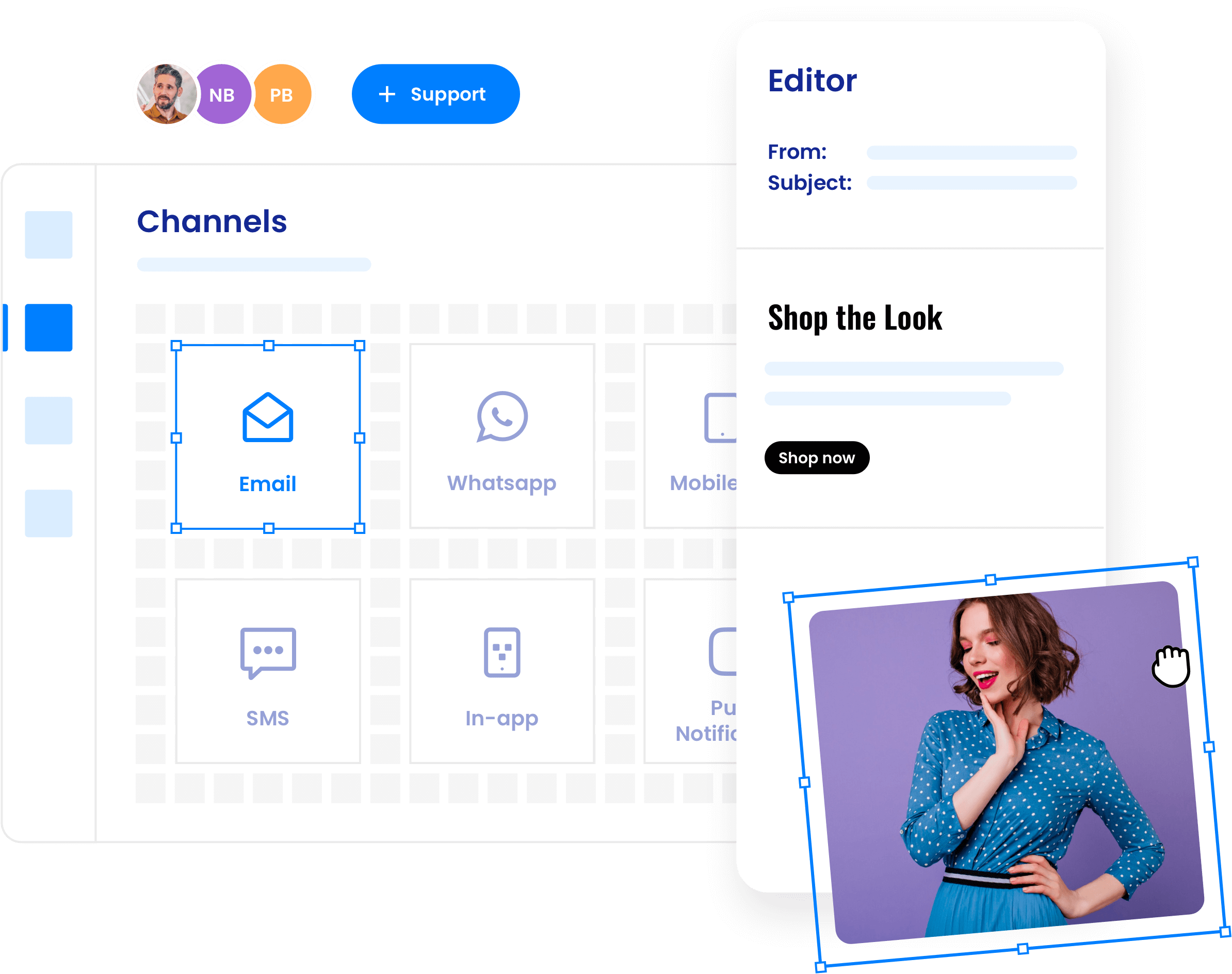Screenshot of a Webpage Interface:

In the bottom right corner of the screen, there is a cropping outline around a small picture of a young lady. The cursor is a hand icon, indicating that the picture can be moved. The young lady appears to be around 20 years old, with fair skin, short brown hair, and makeup. She is wearing a blue dress with polka dots on the top part.

At the top left corner of the screen, there are three icons. The first icon is a small circle featuring a photograph of a white man with black hair, a black beard, and a mustache. The second icon is a purple circle with the initials "NB" in the center. The third icon is an orange circle with the initials "PB" in the center. To the right of these icons, there is a blue, clickable oval labeled "Support."

The main part of the screen displays a large box titled "Channels." Within this box, there are at least six squares, although some may be obscured by an inset. Each square represents a different communication channel. The first square, highlighted with a crop circle, is labeled "Email." The second square, also highlighted, is labeled "WhatsApp." The third is partially obscured but appears to say "Mobile." The fourth square, at the bottom left, is labeled "SMS." The fifth says "In-App," and the sixth is likely "Push Notifications," as indicated by the letters "PU."

An inset is also present on the screen, situated over the main box. At the top of the inset, it says "Editor From:" followed by a blank line, and "Subject:" followed by another blank line. Below these fields, there is text that reads "Shop the Look" followed by two lines of unspecified content. There is a black "Shop Now" button at the bottom of the inset, ready to be clicked.